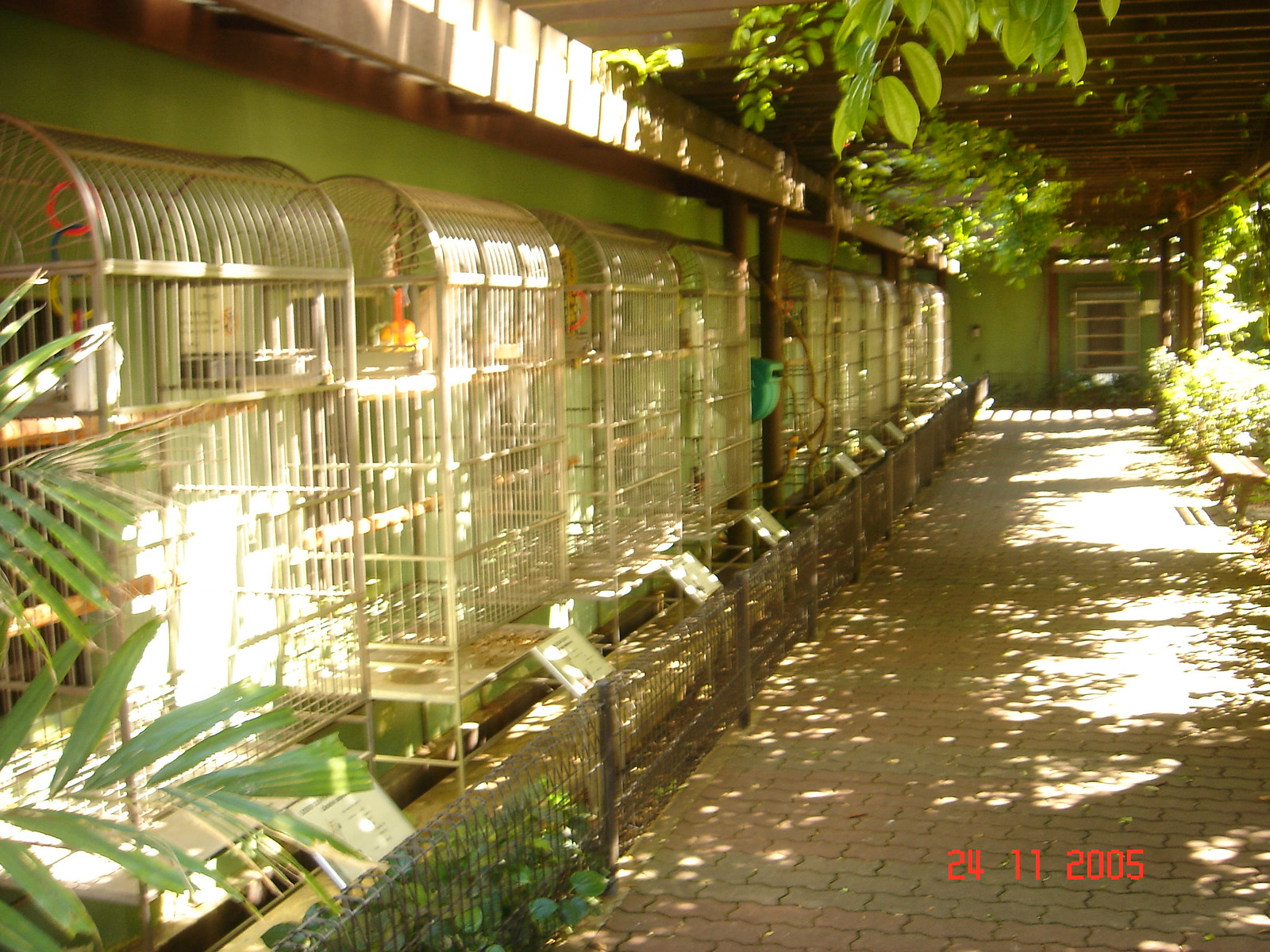This image depicts a somewhat blurry scene of an outdoor area that appears to be part of a garden or an exterior hallway. Along the left side of the image, there is a row of seven white birdcages lined up against a green-painted wall, with various green plants and foliage adorning the space, including climbing up the wall, the ceiling, and scattered around the right side and bottom. The setting seems to be partially enclosed with a deck-style roof overhead, but exposed to sunlight on the right side, indicating it is taken during the daytime. Despite the birdcages being empty, each has a small sign in front of it, covered in plastic. In the bottom right corner, there is a date stamp in red reading "24-11-2005."